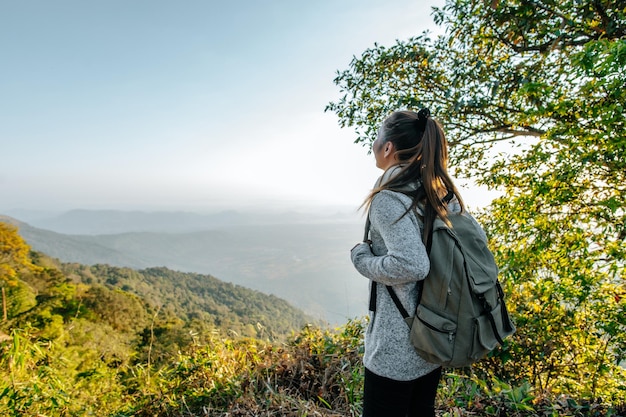The image depicts a young Caucasian woman standing on a scenic overlook, high up on a green, tree-covered mountain, possibly after a hike. She has long brown hair tied in a ponytail and is wearing a gray, hooded sweater with a large backpack that has black straps, along with black pants, possibly workout or running pants. The woman is gazing out into the distance, away from the camera, taking in the beauty of the valley below her which features rolling, fog-covered hills and a hazy sky that transitions from sunny to cloudy. A tree stands to her right, casting some shade, while the rest of the scene is bathed in bright sunlight.